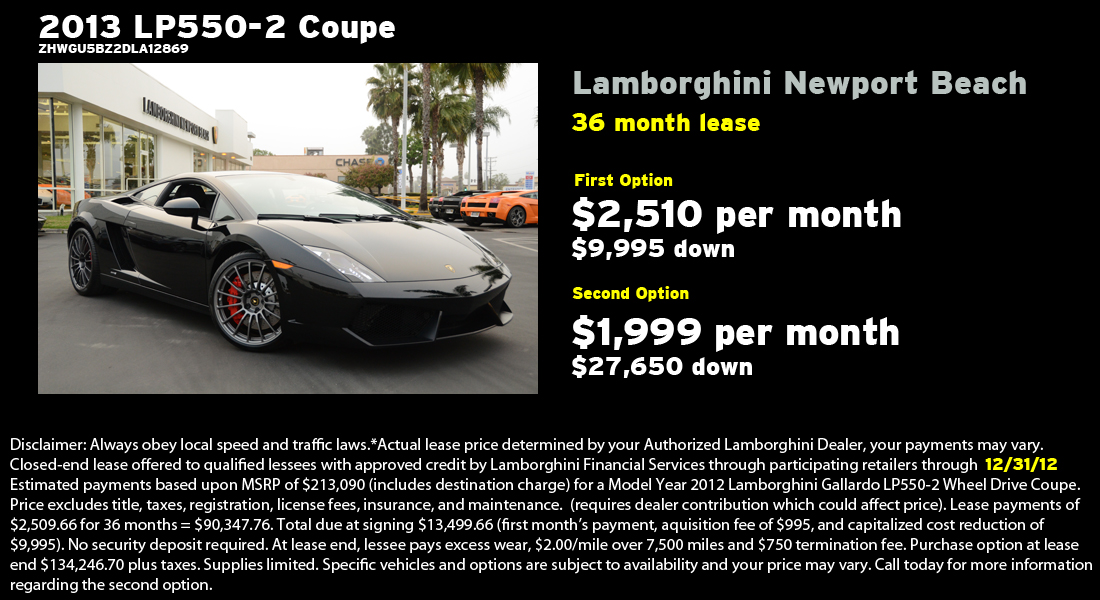The advertisement features a black Lamborghini prominently displayed against a black background, angled toward the bottom right corner of the image. Above the photograph, white text reads "2013 LP550-2 Coupe" with a serial number below. The photo, taken in front of a dealership with other cars visible in the background, highlights the luxurious and sleek design of the vehicle. To the right of the photo, grey text displays "Lamborghini Newport Beach." Below this, in small yellow print, it states the "36 month lease" options: the first option requires $2,500 down and $510 per month, and the second option requires $9,995 down and $1,999 per month. At the very bottom, there is a lengthy disclaimer in white text, providing detailed terms and conditions of the lease agreement. The overall presentation combines color photography with graphic design to create a sophisticated and alluring visual advertisement.